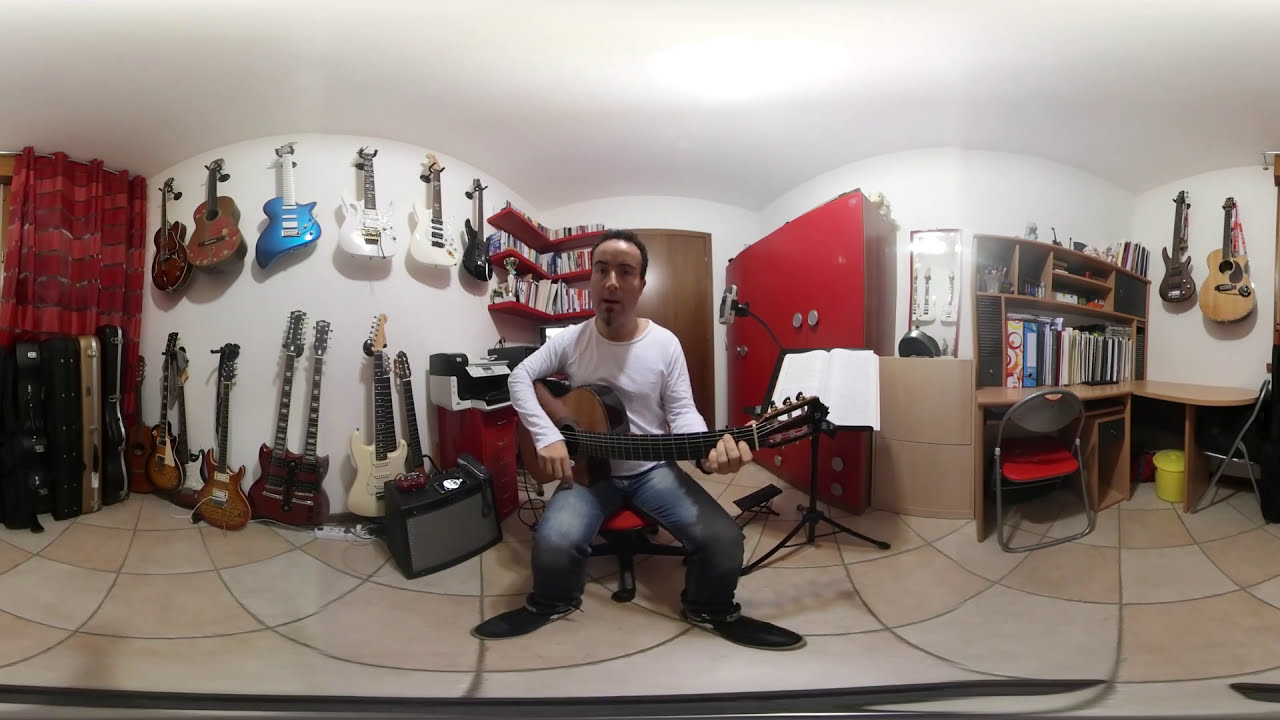A man is sitting in a chair, playing a brown and black acoustic guitar in what appears to be his music studio or guitar collection room. He is dressed in blue jeans, black sneakers, and a white thermal top. He has a small goatee and is looking directly at the camera. The room features white walls adorned with numerous guitars, both hanging from the top portion of the walls and leaning against them. There are multiple guitars visible, including black, brown, red, gold, blue, and white ones, both on the top row and the bottom. Some guitar cases, predominantly black with one gold-colored, are leaned against the left wall next to a red curtain with pink accents.

Directly behind the man is a wooden door, and to his right, there’s a red closet. A brown L-shaped desk with a red cushion is also to his right, along with a black and silver chair. To the man’s left, an amplifier is positioned, and to the far left, multiple guitar cases are stacked against the wall. The floor is tan and tiled. Additionally, a yellow garbage can, a red cabinet, some red shelves holding books, and a music stand with white writing or sheet music are present in the room, contributing to its studio-like atmosphere. The image is captured with a curved fisheye lens, giving it a distorted view and emphasizing the array of musical instruments and equipment.